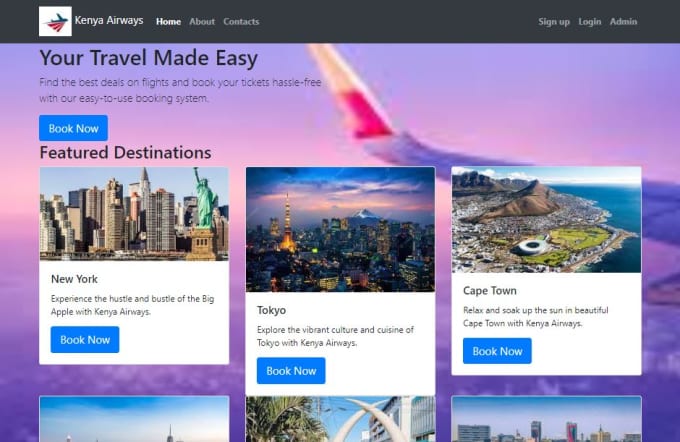The web page features a sophisticated design with a dark gray bezel at the top. At the center of this bezel is a white symbol adjacent to a blue plane adorned with red bands, representing the logo of Kenya Airways. The navigation menu begins with "Home" highlighted in white, followed by "About" and "Contacts" in gray. On the right-hand side, options for "Sign Up," "Login," and "Admin" are displayed.

The background features a vibrant image of a plane in mid-flight, showcasing a gradient tail transitioning from white to red and the edge of the plane wing. On the left side, bold black text declares, "Your Travel Made Easy," accompanied by smaller black text that reads, "Find the best deals on flights and book your tickets hassle-free with our easy-to-use booking system." Below this text is a clickable dark blue button with bold white text that says "Book Now."

Beneath the introductory section, a header in bold black text announces "Featured Destinations." The first image displays the iconic New York skyline with its array of light gray, dark gray, and blue skyscrapers, and the green Statue of Liberty on a dark brown and tan pedestal. Underneath the image, white text reads "New York," while a description in black text invites users to "Experience the hustle and bustle of the Big Apple with Kenya Airways." A dark blue "Book Now" button with white text follows.

Next is an image of Tokyo's skyline, showcasing a variety of towers in orange, green, blue, yellow, and mixtures of yellow and black, with Mount Fuji's snow-capped peak in the background. The sky displays a beautiful gradient of dark blue with bands of pink, orange, and red. In bold black text, "Tokyo" is labeled above a description in black text encouraging travelers to "Explore the vibrant culture and cuisine of Tokyo with Kenya Airways," followed by the same "Book Now" button.

Finally, an image highlights Cape Town, featuring an island with numerous buildings on a large mound resembling a mountain, surrounded by dark blue waters and framed by dark gray and light gray mountains in the distance. The bold black text "Cape Town" precedes a description in regular black text: "Relax and soak in the sun and beautiful Cape Town with Kenya Airways." A clickable "Book Now" button in dark blue with white text is included here as well.

The bottom section of the page features additional photos, although they are partially cut off and not fully visible.